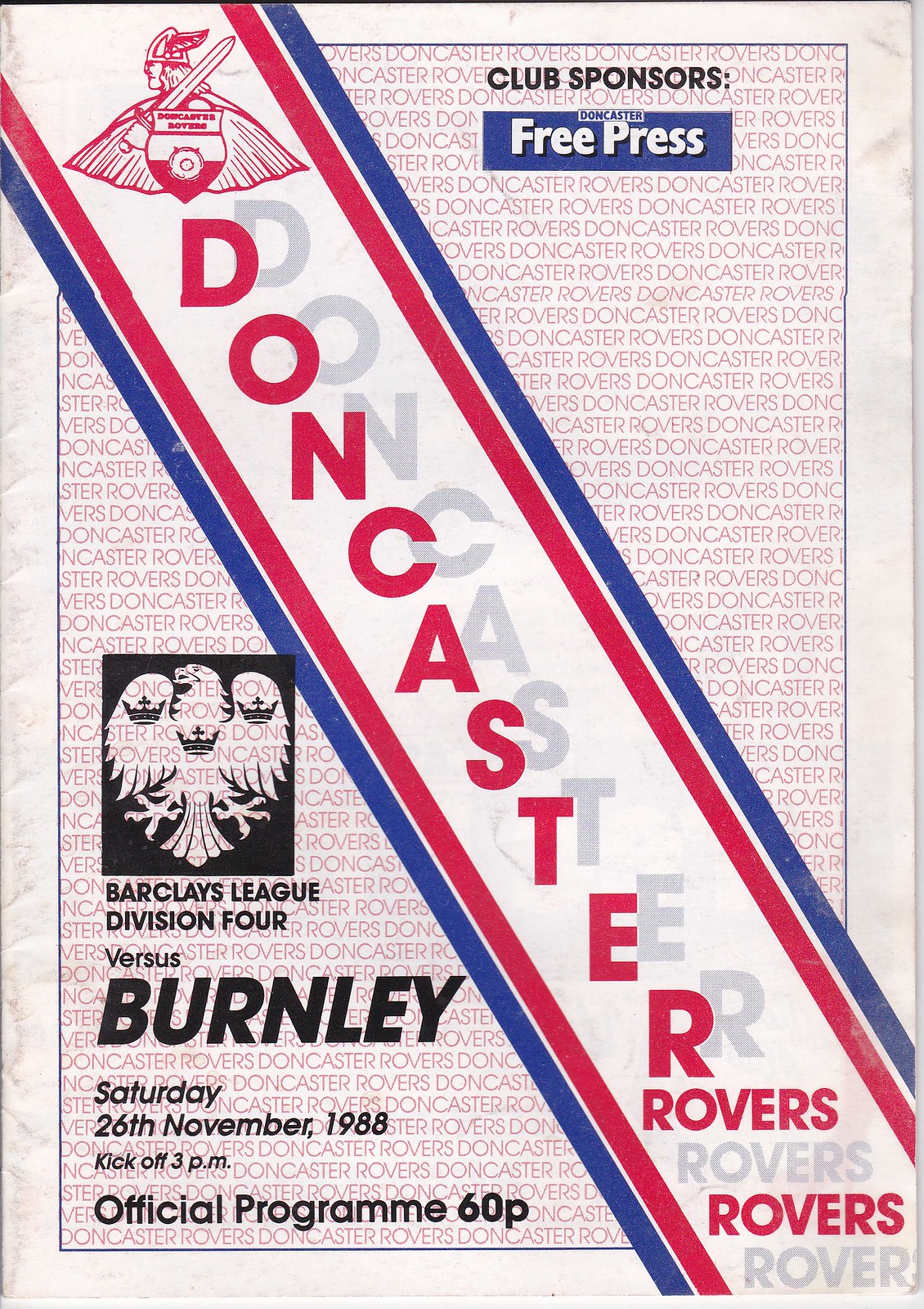The image is an old paper booklet, specifically the front cover of an official program for a Doncaster Rovers football match. The background is primarily white, adorned with a repeated pattern of "Doncaster Rovers" in red text. A prominent feature is a slanted ribbon that runs diagonally across the page from the top left to the bottom right, interrupting the background pattern. This ribbon is flanked by red and blue stripes and contains red text reading "Doncaster Rovers." At the top right of the cover, against a blue background, it states "Club Sponsors: Doncaster Free Press" in white letters. Additionally, at the bottom left, there's text that specifies the match details: "Barclays League Division 4 vs. Burnley, Saturday 26th November 1988, Kick-off 3 p.m." Below this, it reads "Official Program" and "60p." A crest depicting a Viking with a shield and cape, symbolizing the Doncaster Rovers, is also featured prominently.